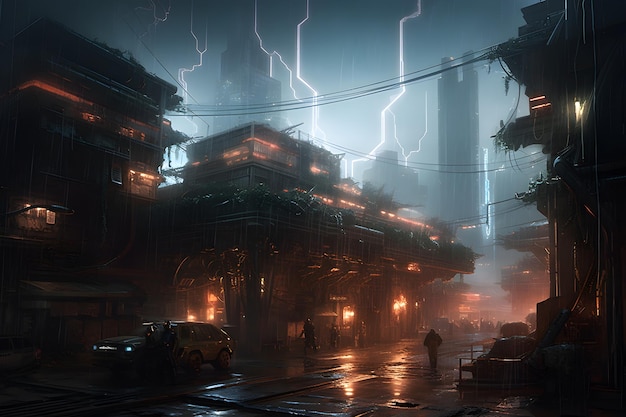The photograph showcases a night scene in a futuristic, dystopian city engulfed in a powerful thunderstorm. Sky-high lightning bolts dramatically illuminate the dark, rain-soaked streets, creating a striking contrast against the towering skyscrapers in the background. The wet ground reflects the orange city lights, adding a surreal glistening effect to the urban landscape. 

In the foreground, the area appears run-down and dominated by lower buildings, with power cables stretching between them. A lone car is parked on the street, while a solitary man walks down the middle of the road amidst numerous scattered puddles. On the sidewalks, people are seen braving the downpour, some crossing the street, while others in the distant background seem to be lined up, possibly near a train station inferred from the darker, less illuminated part of town. The entire scene is bathed in the eerie, intermittent flashes of lightning that highlight the jagged edges of the stormy sky, adding to the dystopian and futuristic atmosphere.